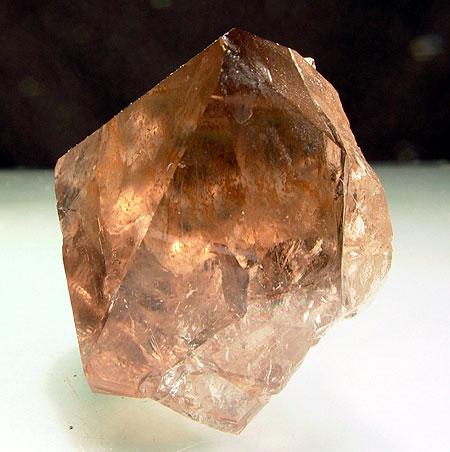This image depicts a sizable, irregularly shaped gemstone or possibly an amber rock, resting prominently on a pristine white surface against a solid black background. The rock, approximately the size of a person's fist, boasts a rich palette of brown and golden hues, transitioning through various shades from light, almost translucent amber to dark, deep browns and near-black tones. Its surface features a mix of sharp edges and smooth sides, with certain areas seemingly shaved or cut to create multiple facets that catch and reflect the light. Some sections of the stone appear clearer, allowing light to penetrate, while others remain distinctly opaque. The object, centrally positioned in the image, could be a part of a collection, either in a museum or owned by an avid collector. There are no text or additional items present, emphasizing the raw, natural beauty and intricate details of the gemstone.